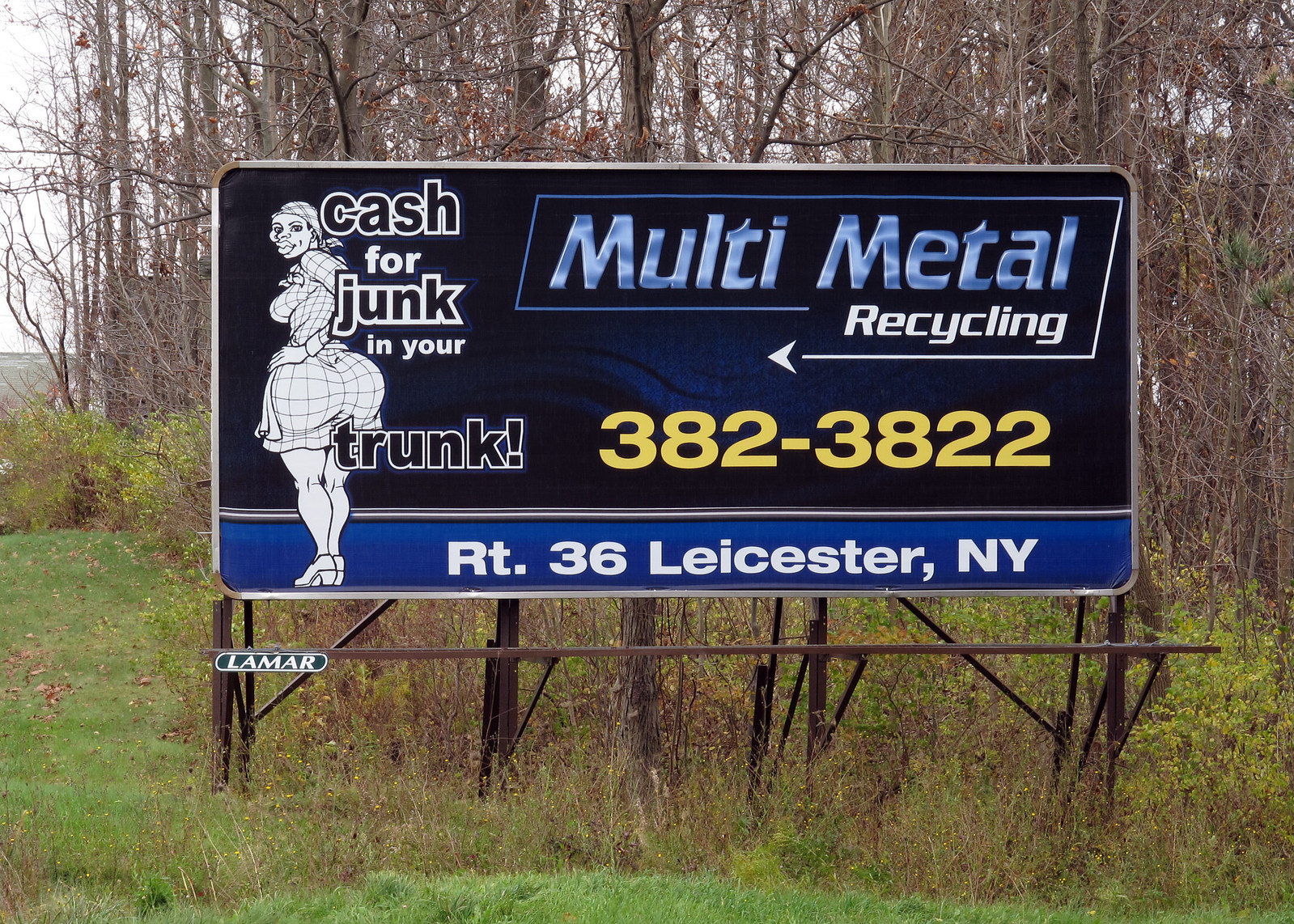This is a detailed caption for the image described:

"A roadside billboard advertising Multi-Metal Recycling catches the eye with bold text encircled by an arrow. The arrow encircles the words 'Multi-Metal Recycling' and points towards a cartoon character on the left side of the billboard. The character, a woman with a prominent posterior, stands with one hand on her hip and glances back over her shoulder. Accompanying her image is the cheeky slogan 'Cash for Junk in Your Trunk.' A vivid blue strip runs along the bottom of the sign, bearing the text 'Route 36, Leicester, New York.' Additionally, a smaller, green sign with white text reading 'Lamar' is situated at the bottom left corner of the billboard."